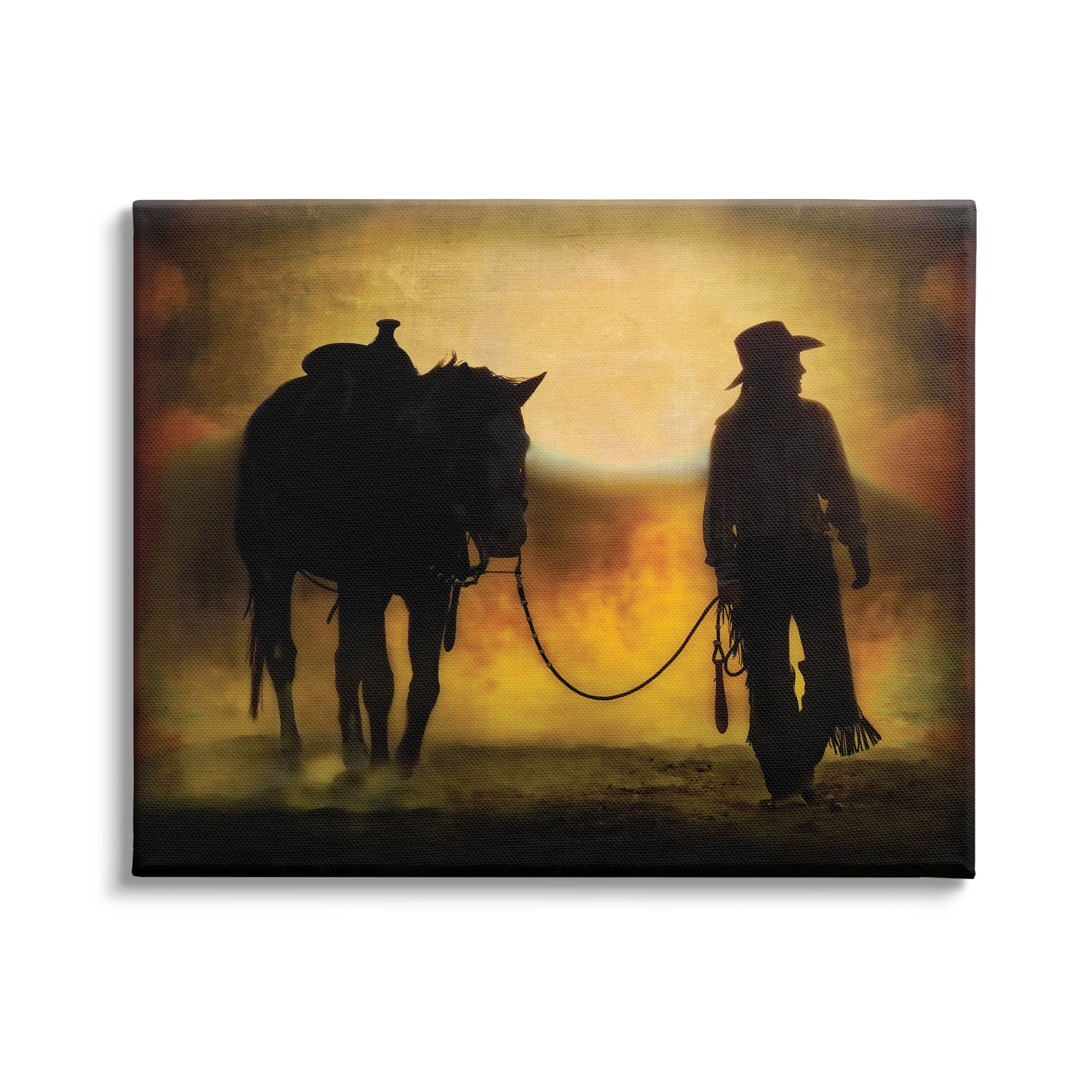This is a detailed painting on a canvas print featuring the dark, silhouetted figures of a horse and a cowgirl walking together. The horse, positioned on the left side of the canvas, is slightly angled to the right and dons a prominent saddle and bridle. Attached to the bridle is a rope held by the cowgirl, who occupies the right side of the painting. She is dressed in dark fringed pants, a long-sleeved shirt, and a cowboy hat, looking ahead to the right. The background is a blend of colors: a light blue horizon transitioning into a vibrant orange and yellow sky with smudged orange, brown, and gray clouds framing the scene. The bottom of the canvas depicts a dark brown, almost dirt-like ground. Despite the darkness of the figures, the painting captures a sense of motion and interaction between the cowgirl and her horse.